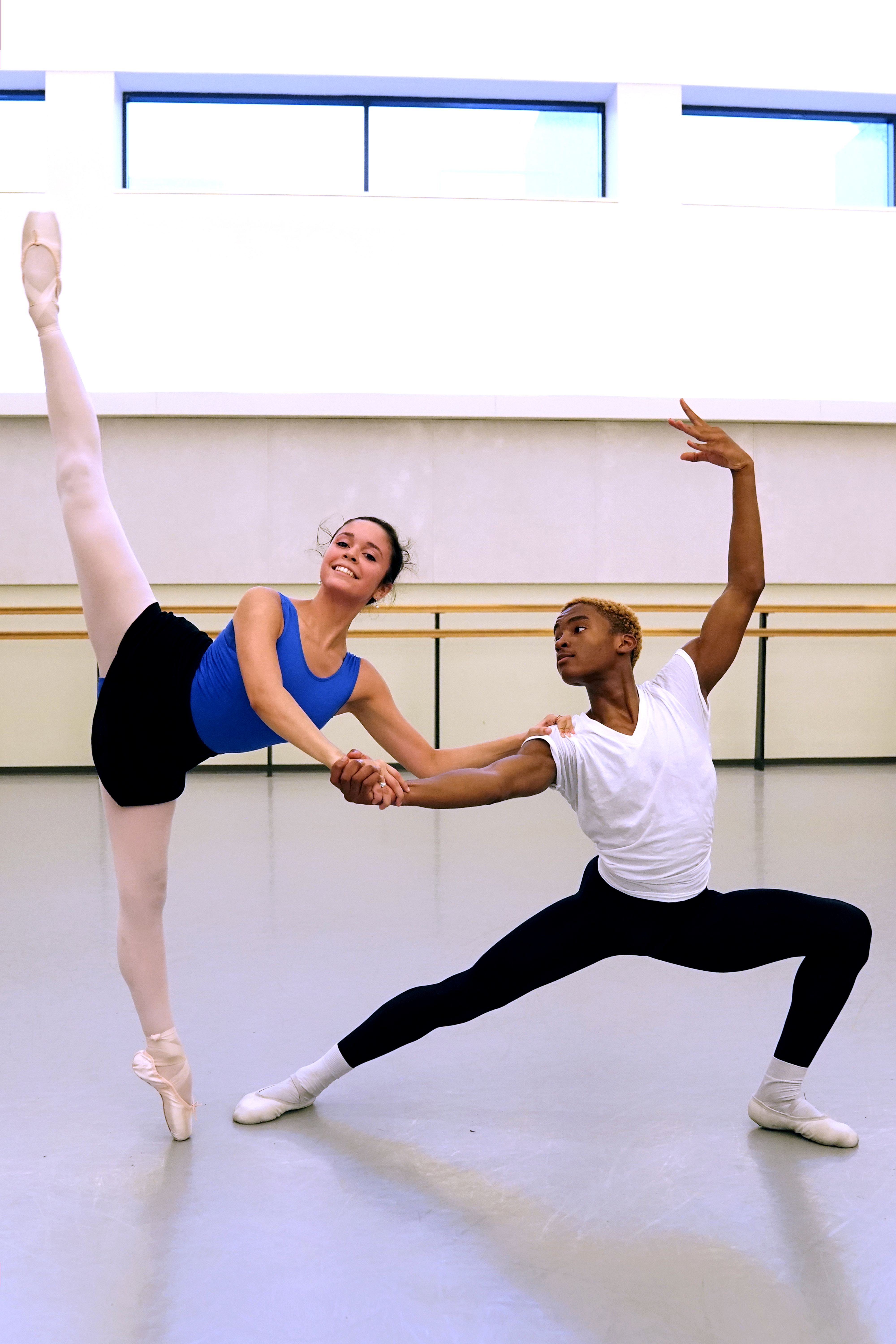In this photograph, two dancers are captured in a brightly lit dance studio with large windows that flood the room with natural light. Both dancers strike a poised, intricate pose on a light gray or white dance floor. The dancer on the right is a man with dark skin, wearing a white cotton T-shirt, black leggings, white socks, and white ballet shoes. He is performing a graceful warrior-like pose with his left arm raised high and his right arm extended towards the woman on his left. His stance shows one leg bent at the knee and the other extended straight behind him at a 45-degree angle. 

The woman on the left, who has light skin and her hair styled in a ballerina bun, exudes elegance as she balances on her toes on one leg. She wears a blue top and a short black skirt with white tights and white or pale pink ballet shoes. Her other leg is raised high in the air, almost in a full split. She holds her partner’s outstretched right arm for support while smiling directly at the camera. Behind them, a yellow railing with black bases lines the white background, adding structure to the studio setting. The synergy and focus between the two dancers are palpable, making this an exquisite capture of grace and coordination.